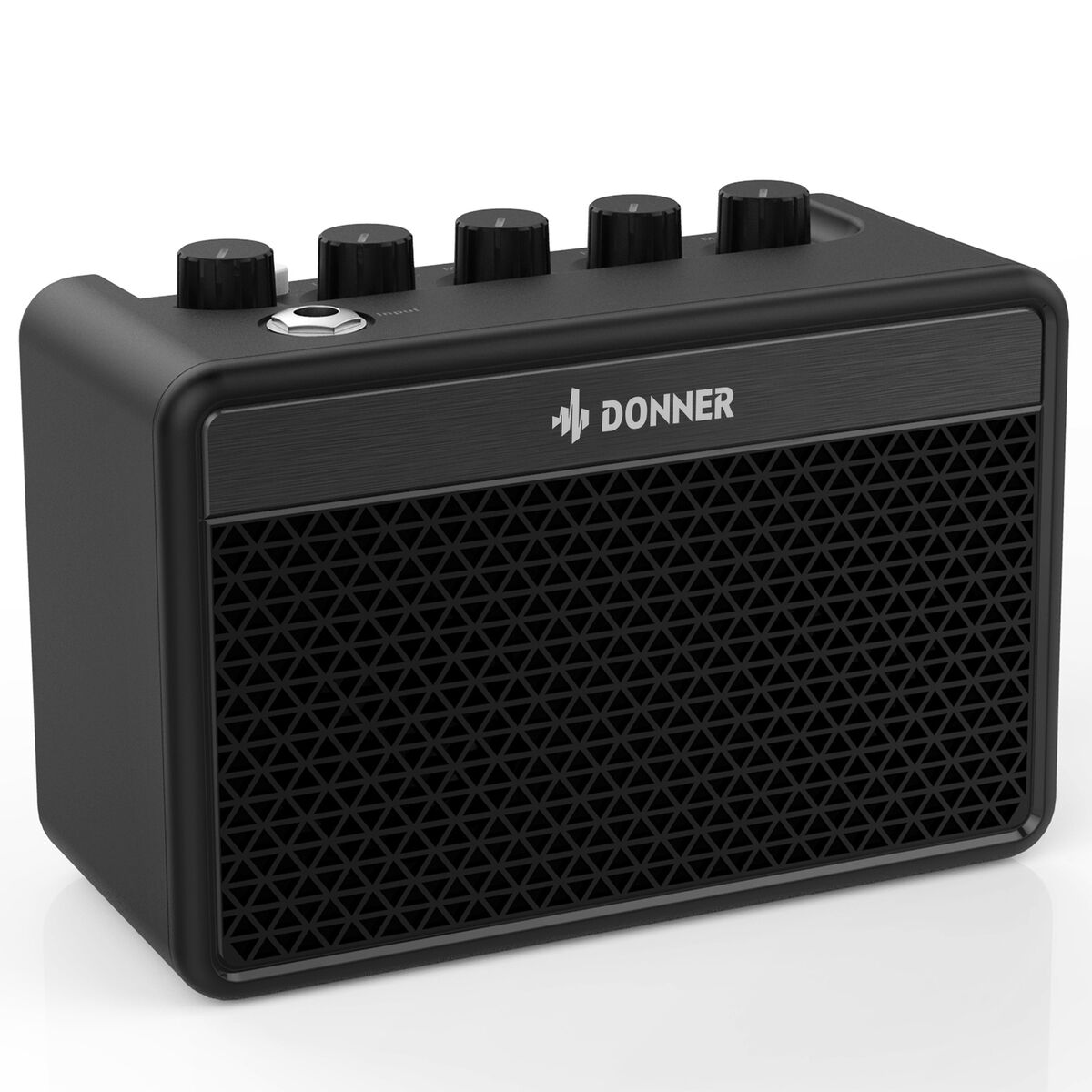The image showcases what seems to be a small audio amplifier or speaker unit, positioned against a white background, making it an ideal advertising or promotional photo. The device is basically a rectangular box, predominantly defined by its speaker grill, which features a diamond-patterned design occupying about 80% of the front-facing surface. Above this grill, there's a black, matte-finished horizontal bar that displays the brand name "Donner" in white text, and to the left of the brand name, there is a small squiggly line or signal emoji. The top panel of the unit houses five recessed black knobs arranged in a straight line, presumably for adjusting various audio settings; however, the exact labels on these knobs are not visible. Additionally, there is a silver input jack situated to the left of these knobs, suggesting potential use with a guitar or other audio input device. The overall color scheme of the unit is a greyish-black, providing a sleek and modern appearance.